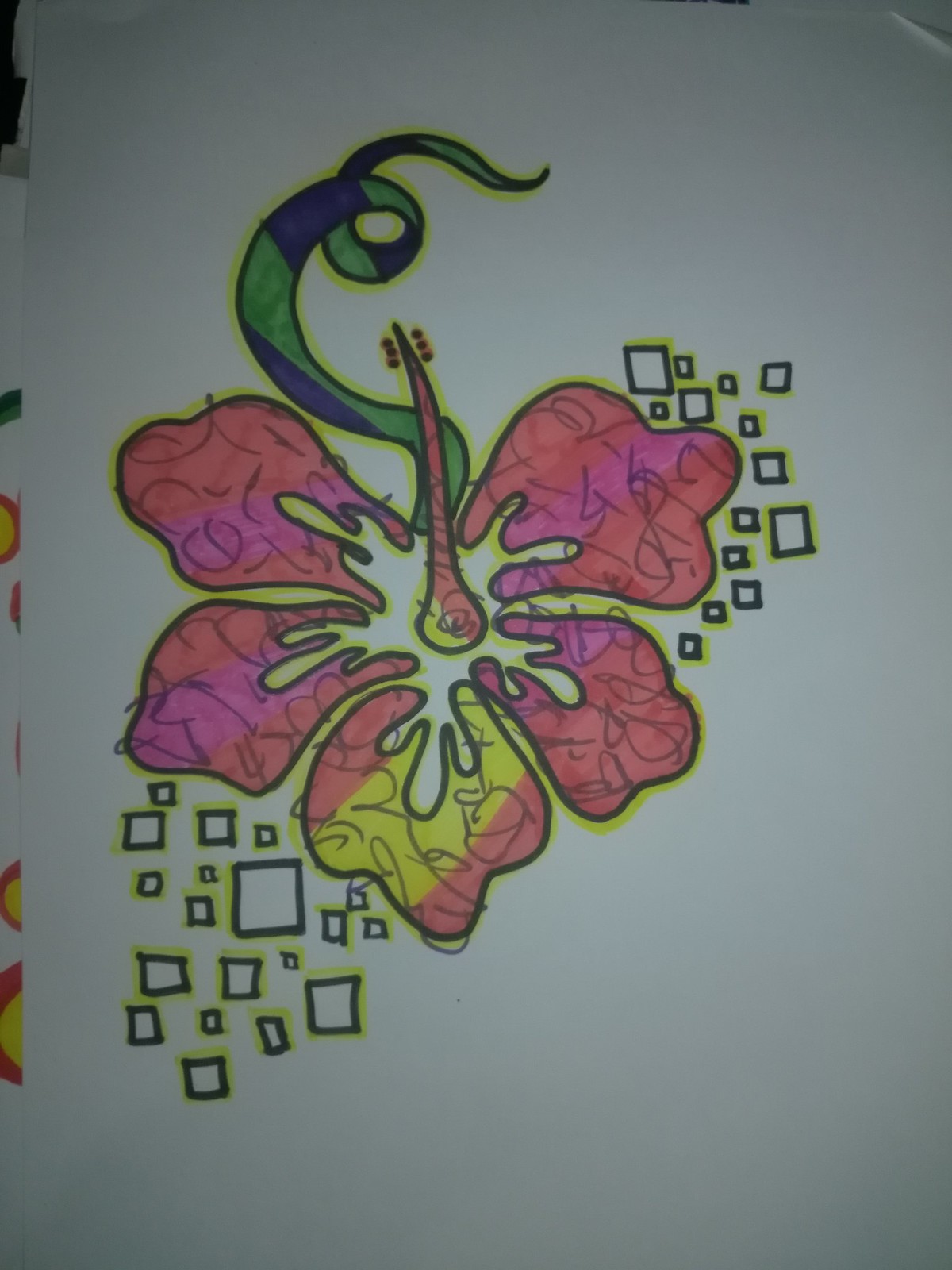This image depicts a stylized flower icon, showcasing an intricate doodle design. The flower features five pinkish petals, each accented by splashes of color that radiate from the center. The petals are adorned with small yellow highlights framed by black trim, situated on two sides of each petal. From the center of the flower, a slender, upward-pointing stem with subtle ridges emerges. Additionally, a larger, curly stem-like structure extends from the flower, rendered in light green and blue hues, adding a whimsical touch to the overall design.